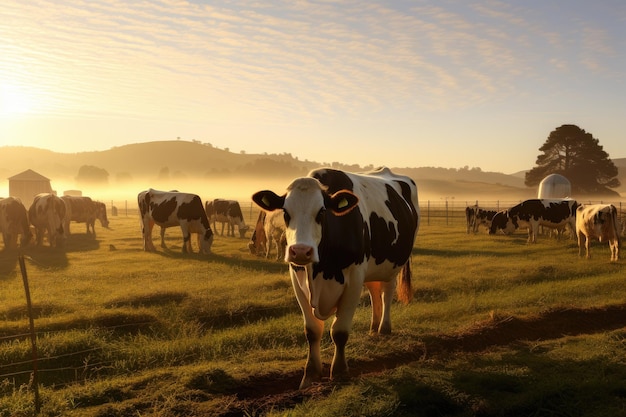In this vibrant outdoor scene, the focal point is a large cow with a white coat adorned with dark brown spots, standing still and gazing directly at the photographer. His prominent size is accentuated by his position in the foreground, with curious brown ears jutting out to the sides as if he’s listening intently. Surrounding him, a herd of black and white cows are scattered across a lush, enclosed pasture, some contentedly grazing on the abundant grass while others group together. A gray wire fence stands in front of the foreground cow, encapsulating the peaceful setting. The background reveals rolling hills dotted with green trees and bushes, under a beautiful, partly cloudy blue sky. In the far left corner, a shed or barn peeks out, accompanying a grain silo and another round-topped silo emitting wisps of steam in the cool morning air. The pastoral landscape, enriched with rustic structures and framed by nature's beauty, suggests a serene, early morning on a picturesque ranch.